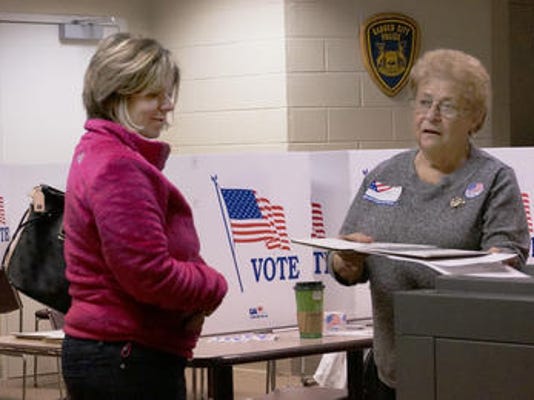The image captures a detailed scene inside what appears to be a voting poll booth, possibly doubling as a campaign headquarters. Two women stand at the center of the photograph; the woman on the left, clad in a purply fuchsia jacket and dark jeans, has shoulder-length dark brown hair and carries a black handbag. She faces toward the woman on the right, who sports a gray shirt adorned with flag stickers and wears spectacles. The right woman appears older and is assisting the other in what seems to be the balloting process, possibly with a ballot box visible at the lower right corner.

Behind them, the background features white walls with a tiled pattern and a yellow and blue shield. A door and cinderblock walls painted cream also frame the scene. The space is dotted with several signs and banners, most notably showcasing the American flag and the text "VOTE" in bold blue letters. A green disposable coffee cup emblazoned with the word "VOTE" is placed on a table between the women. Nearby, additional voting booth partitions made from cardboard carry the same patriotic theme with red, white, and blue colors. Stickers and a variety of campaign materials further litter the area, adding to the active and organized atmosphere of civic engagement.